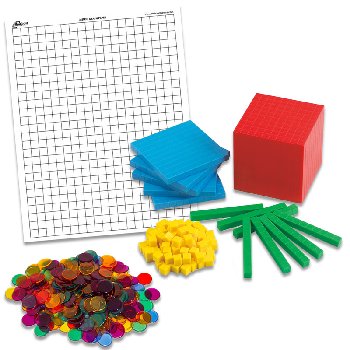This detailed image showcases a collection of educational math tools commonly used in schools. The background features a white page printed with a grid of small, one-centimeter square outlines, some of which appear to be missing, giving it a slightly maze-like appearance. Neatly arranged on top of this grid paper are various counting blocks and chips in vivid colors. 

To the left, there's a mixed pile of round, translucent counting chips in colors such as purple, turquoise, pale blue, yellow, light green, and red, resembling flattened plastic circles about the size of pennies. 

Adjacent to the chips are small yellow square blocks, each measuring 1 cm by 1 cm. Next to the yellow blocks lies a series of longer, green strips, each composed of 10 small blocks joined together. 

An arrangement of larger, square blue blocks, assembled into a 10 by 10 grid to form 100 blocks, sits further to the right. 

Dominating the center is a red cube made up of 1,000 smaller blocks, illustrating a perfect cube structure. These colorful blocks and chips are clearly organized for visual and tactile counting exercises, ideal for helping children understand numerical values and arithmetic concepts.